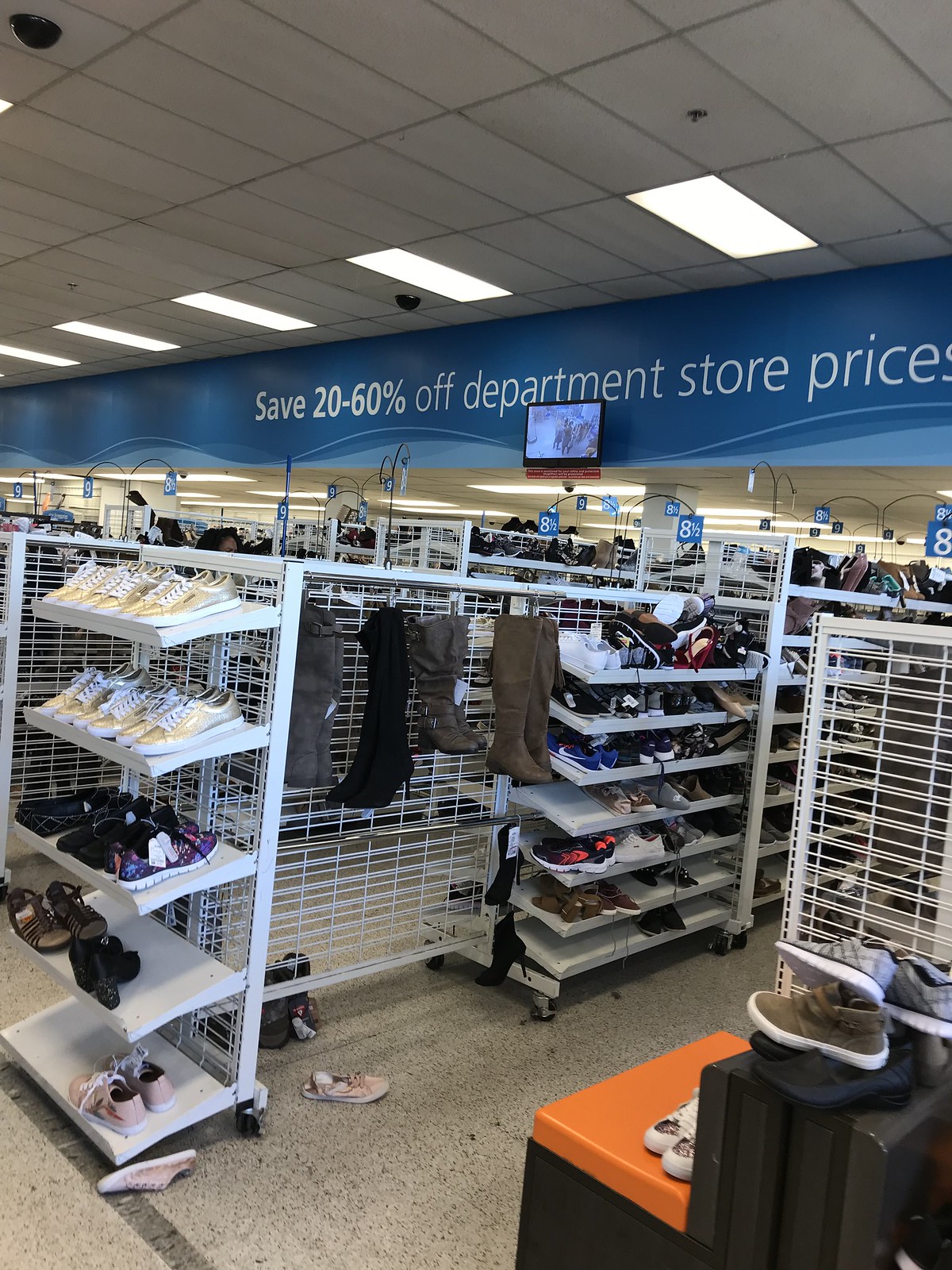Inside what appears to be a department store, the scene features a white tiled ceiling adorned with light fixtures running across its length. A visible security camera is mounted on the top left corner, overseeing a portion of the store. At the far end of the store, a prominent blue banner spans the width of the image, advertising "Save 20-60% off department store prices" in bold lettering. 

A TV monitor displaying the live feed from the security camera serves as a reminder of the store's surveillance. The store's floor is cluttered with scattered items, including shoes and various articles of clothing. The shelves, which are made of a white metal and slightly sloped downward, are lined with an assortment of footwear such as shoes and boots. These shelves also feature markings indicating shoe sizes, notably displaying sizes 8.5 and 9. 

The overall organization of the store appears to be haphazard, with items strewn about and different lanes forming aisles through the space.